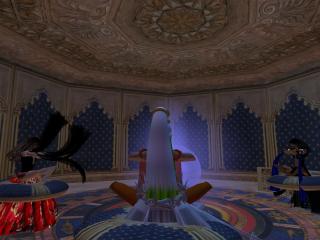The screenshot from the video game depicts an intricately designed, oval-shaped room with a highly decorative roof characterized by golden and maroon mandala-like patterns, along with a large star shape at the center featuring white points. The ceiling transitions into fringed beige, with light brown curtains hanging in U-shapes around the top perimeter. The walls are a striking blue with dark and light gray trim, adorned with small white designs. Dominating the room is a blue carpet decorated with pink and yellow circular designs. A figure with dark brown skin, sitting cross-legged and facing away from the camera, is positioned in front of a glowing purple object. To the left is a blue table with a black item on a red base, while another blue table with a character is slightly visible to the right. The dimly lit ambiance and the intricate elements create a richly detailed and almost mystical environment.